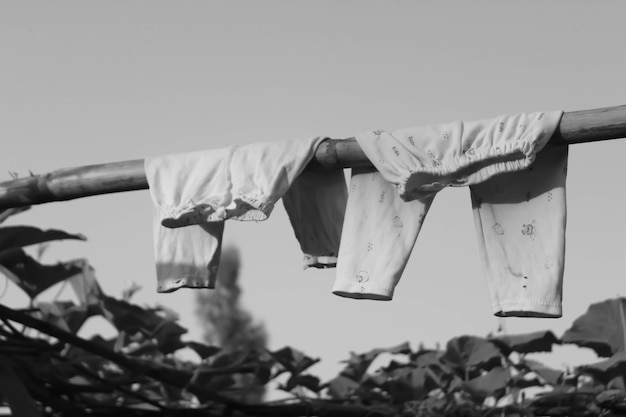In this high-quality black-and-white photograph, two pairs of pants, reminiscent of old-style stretch pants or bloomers, are draped over a thick bamboo pole that runs horizontally across the middle of the frame. The pants, possibly designed for females due to their thin and ornate patterns, vary in size with the one on the left appearing smaller and more delicate, while the one on the right boasts a thicker waistband and longer legs. The sky above is a consistent gray, a likely artifact of the monochrome filter. Below the bamboo pole, the ground is densely covered with dark foliage, perhaps leaves or flowers. In the distance, slightly off-center to the left, a large tree silhouette is visible, further accentuating the outdoor setting of the scene. The overall brightness suggests it is daytime, despite the grayscale presentation.